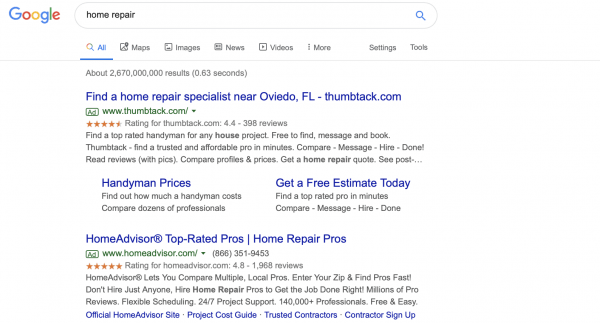This image is a screenshot of Google search results for the query "Home Repair." In the top left corner, the Google logo is clearly visible, and to its right, there's a search bar containing the text "Home Repair." Underneath the search bar are various clickable options including All, Maps, Images, News, Videos, and more. The search results displayed below feature the first result titled "Find a Home Repair Specialist Near Ovadio, Florida" from Thumbtack.com. The second result is "Home Advisor Top Rated Pros, Home Repair Pros" from HomeAdvisor.com. Each of these search results includes a brief description of the respective website and its services. The page has a white background, providing a clean and straightforward layout typical of Google search results.